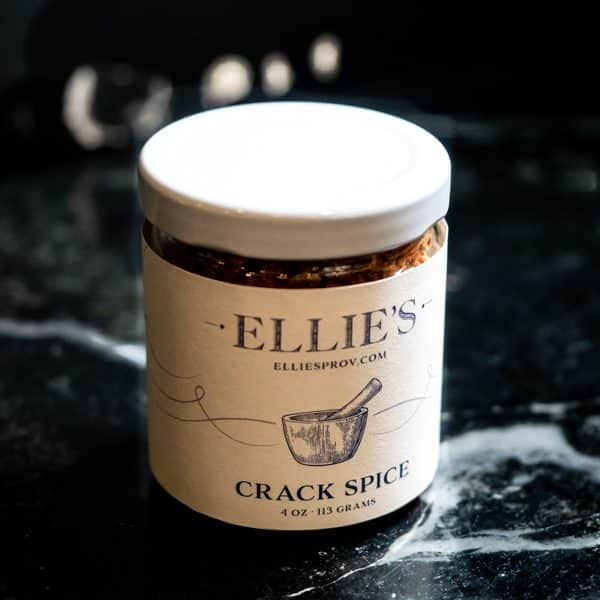This professional product image features a clear, cylindrical glass jar with a white plastic or metal lid, prominently displayed on a sleek black marble surface with white veining. The jar contains a reddish-brown mixture, identified as "Ellie's Crack Spice." An off-white label encircles the jar, detailed with a blue curved line design. The label includes the brand name "Ellie's," followed by the website "elliesprov.com" and a black and white illustration of a mortar and pestle. Further down, the label specifies the product as "Crack Spice" and notes the quantity as four ounces (113 grams). The photograph, taken with a shallow depth of field, highlights the jar sharply while subtly blurring the background, lending a professional and focused aesthetic suitable for a storefront or online marketplace.